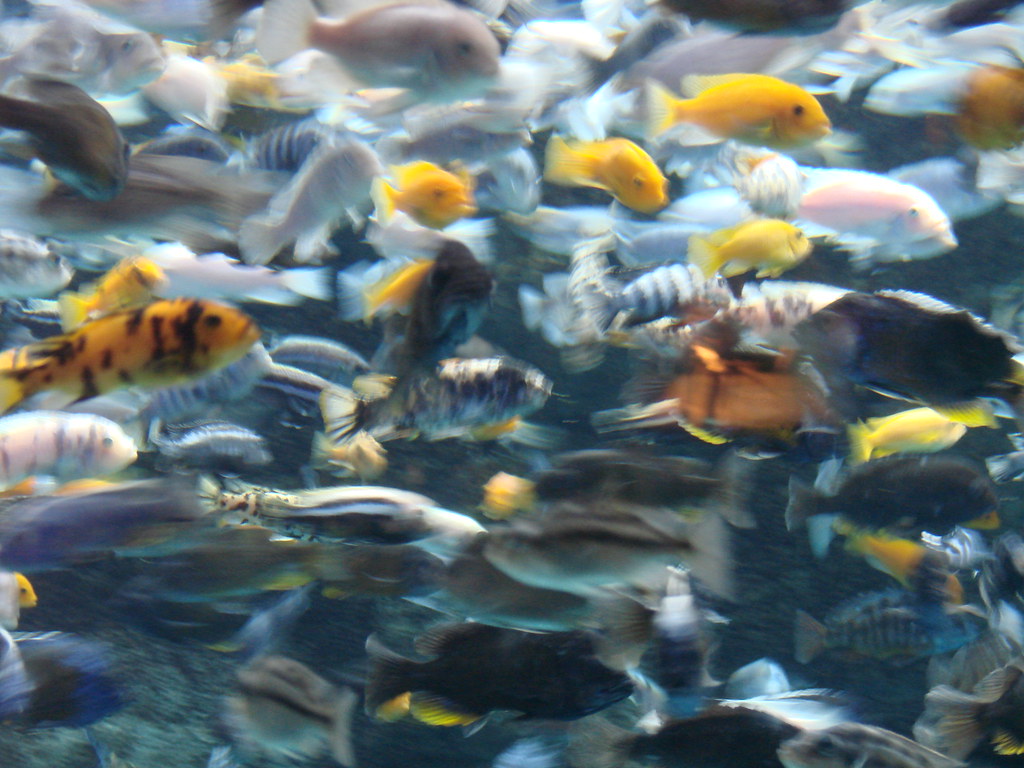The photograph showcases a bustling fish tank teeming with a variety of fish. Dominating the scene are numerous vibrant yellow fish, some adorned with distinctive black spots and stripes, and a mix of light and dark yellow baby fish. Also present are a multitude of white fish, appearing somewhat blurred, suggestive of their rapid, energetic movements. Among the clear and colorful swimmers, there are also several dark blue fish, one notably featuring a yellow tail. The blue water creates a serene backdrop, contrasting with the lively traffic jam of fish primarily swimming from left to right, though some appear to be changing direction. In addition to the predominant yellow and white fish, spots of orange, black, grey, and pink fish add to the rich variety. The tank bottom features corals or rocks, enhancing the naturalistic setting of this aquatic scene.